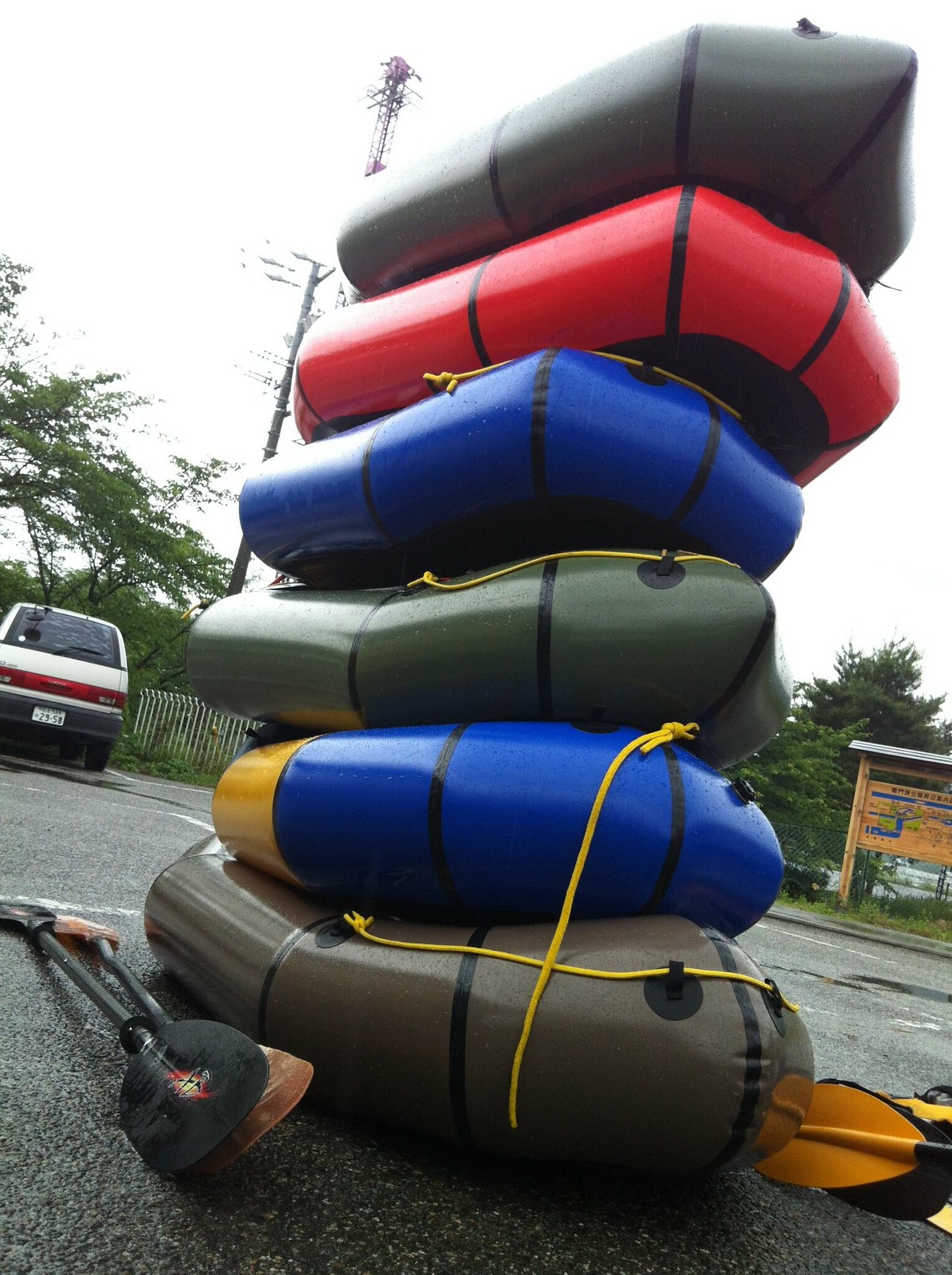This photograph, taken in an outdoor parking lot, captures a stack of six inflatable alpaca rafts piled one on top of another. The bottommost raft is brown and curved at the top, providing a base for the rest. Sitting atop the brown raft is a blue and gold raft, followed by an olive green one, another blue raft with a yellow rope, a red raft with black striping, and finally, a grayish-green raft with a pointed shape on the very top. Surrounding the stack of rafts are several paddles in black, brown, orange, and yellow, scattered on either side on the ground. In the background, a white car is parked near a fence, with trees providing a natural backdrop. The primary focus of the image is the intricately detailed stack of rafts and the paddles lying beside them.